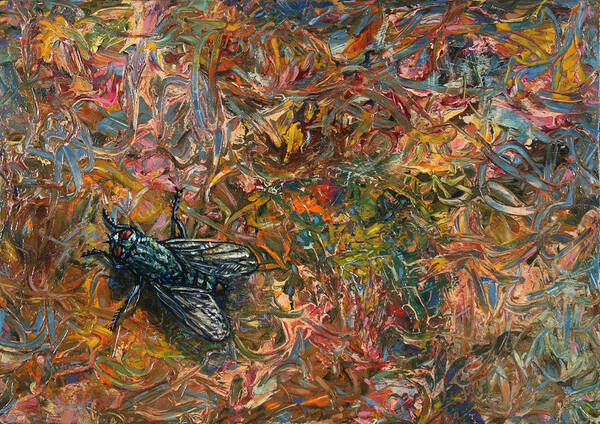This vibrant and dynamic painting features an abstract background composed of swirling and interlocking smears and curves of nearly every imaginable color, including blues, greens, oranges, yellows, pinks, reds, grays, blacks, and whites. The energetic application of paint, resembling a style akin to Jackson Pollock, showcases the artist's action and motion, creating an overall bright and colorful scene without much use of black or heavy shadows. Amidst this colorful chaos, a striking focal point emerges in the bottom left quadrant: a very large, greenish, hairy fly with prominent red eyes. The fly, taking up about 10% of the canvas, appears at rest, with its face directed towards the top left corner of the painting. Despite the abstract nature of the background, the fly stands out as the only recognizable form, anchoring the piece with its detailed depiction. There are no visible signatures on this painting.